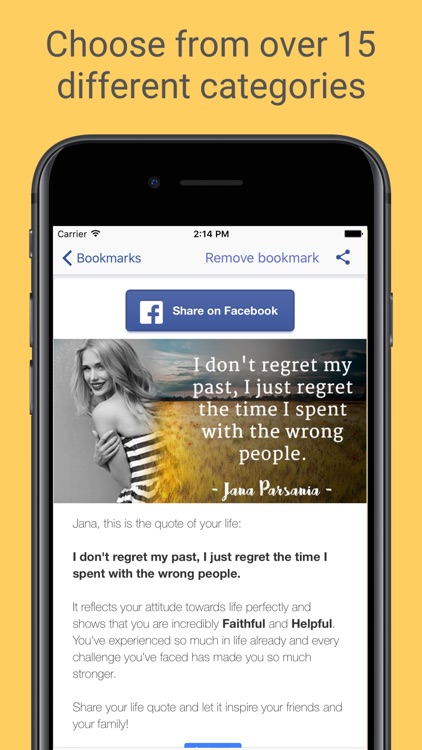The image is a promotional screenshot for a mobile app, presumably designed for sharing inspirational quotes. At the top of the screenshot, text reads: "Choose from over 15 different categories." The centerpiece of the image is an iPhone display. 

Towards the middle of the phone screen, there is a prominently placed button that says "Share on Facebook." To the left of this button, there is a quote displayed in a stylish font: "I don't regret my past, I just regret the time I spent with the wrong people." Beneath the quote, the name "Janna Parsinia" is listed, attributed as the author. 

Further down, a message addressed to Janna reads: "Janna, this is the code of your life." Immediately following this, the same quote is repeated, accompanied by a detailed analysis: "Reflects your attitude towards life perfectly and shows that you are incredibly faithful and helpful. You've experienced so much in life already, and every challenge you face has made you so much stronger. Share your life quote and let it inspire your friends and your family." 

The words "faithful" and "helpful" are bolded for emphasis. This design and text collectively suggest a focus on personal growth and the power of sharing one's life experiences to inspire others.